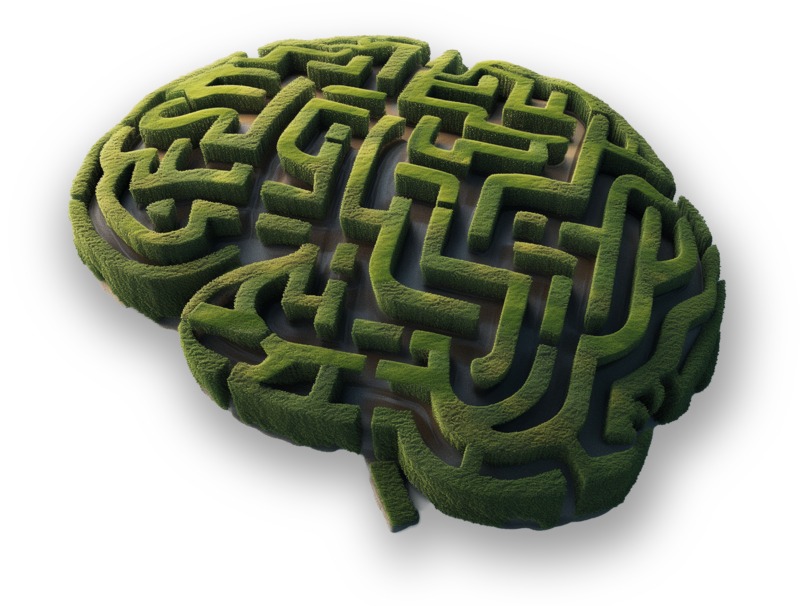The image is a detailed 3D color illustration featuring a complex green maze designed to resemble the shape of a human brain. The green hedgerows forming the maze are intricately trimmed, giving them a raised, three-dimensional appearance that stands out against a plain white background. The maze appears to float, with a slight shadow effect accentuating its three-dimensionality, particularly toward the bottom and right side. The orientation of the illustration is landscape, measuring approximately four inches wide and three inches high, with the brain shape slightly tilted so that the left-hand corner is higher than the right-hand side. The entrance to the maze is located at the bottom center, where the spinal cord would typically attach. Notably, the green of the hedges varies in color—brighter and yellowish on the left and darker on the right. The ground within the maze transitions from a lighter tan brown to a darker gray, adding depth and realism to the illustration.